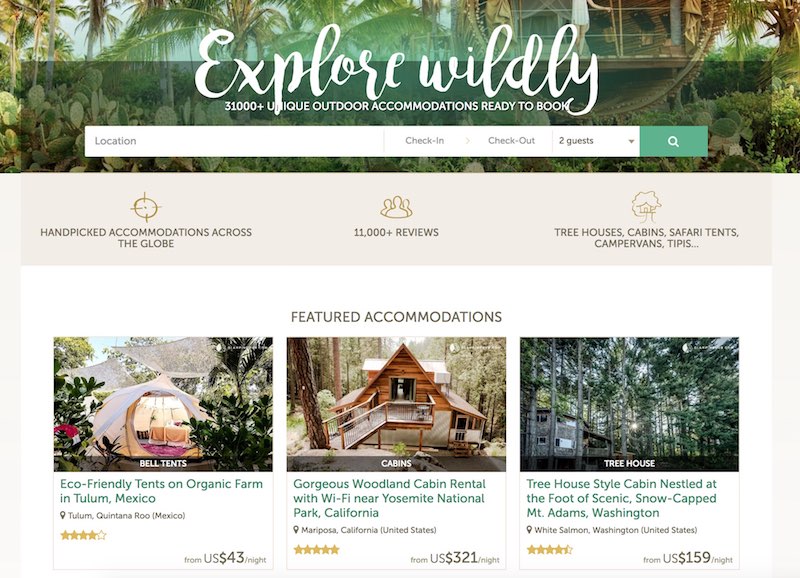The image showcases a vibrant website designed for booking unique outdoor accommodations, promoting the tagline "Explore Wildly." Highlighted at the top is a prominent search bar allowing users to input their location, check-in and check-out dates, and specify the number of guests. This bar features a green search icon encircling a magnifying glass.

Behind the search interface is an inviting tropical scene, complete with lush foliage and towering palm trees typical of a tropical island. A woman clad in a short white dress is pictured amidst the greenery, adding a sense of adventure and relaxation to the scene.

Below the main image, the website emphasizes its hand-picked accommodations across the globe, boasting over 11,000 reviews. Accommodation types include tree houses, cabins, safari tents, camper vans, and teepees.

Further down, the "Featured Accommodations" section presents several enticing options. The first is a colorful bell tent with a beige exterior and vibrant pink and orange interior, described as eco-friendly and located on an organic farm in Tulum, Mexico. Next is a stunning wood cabin with Wi-Fi, available for rental near Yosemite National Park in California. The last highlighted option is a treehouse-style cabin nestled at the base of the picturesque, snow-capped Mount Adams in Washington.